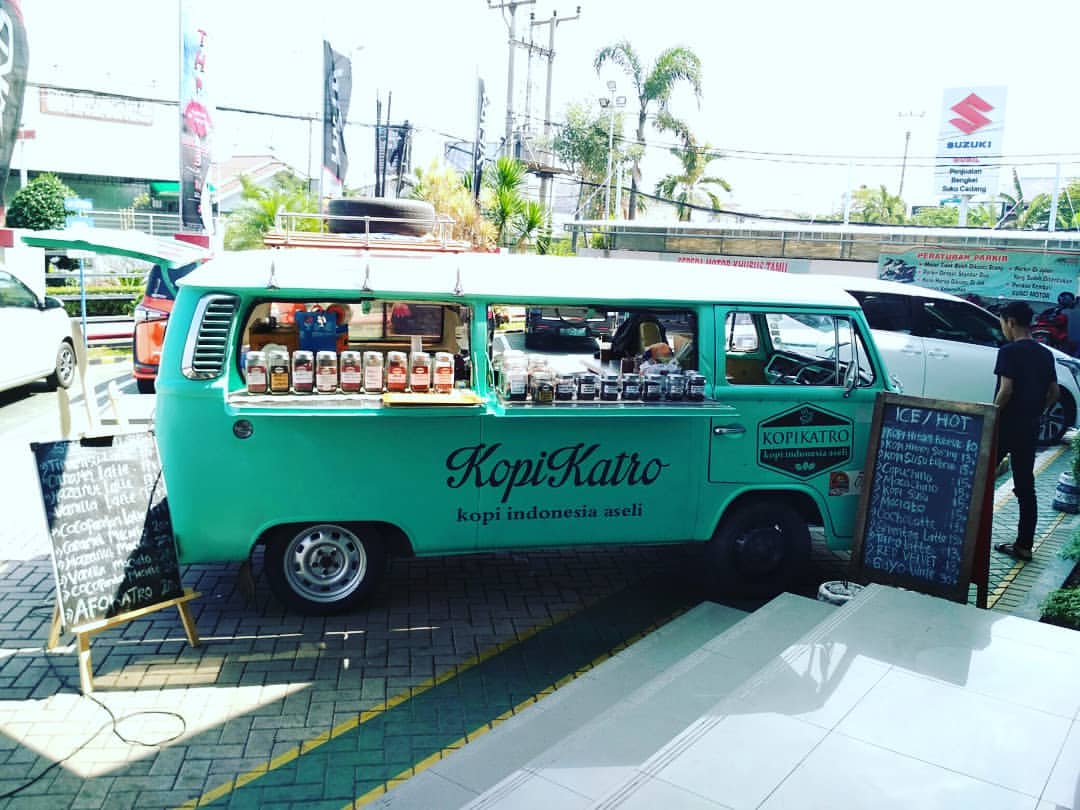In the center of the image, there is a vintage, light teal food van facing to the right, parked on a gray, brick-patterned ground. The van has its windows open, forming shelves that display various jars, likely containing different types of coffees such as cappuccinos and lattes. Above the windows, the name "Kopi Katro" is prominently written in black letters, with the tagline "Kopi Indonesia Aseli" underneath. 

In front of the van stands a man in black pants and a black short-sleeved shirt, facing away from the viewer and looking down at the sidewalk. A chalkboard with a brown frame is placed outside the van, displaying a menu written in white chalk, with the words "Ice/Hot" followed by a list of items and their prices.

The background of the photo includes power lines, trees, and a light blue sky with some white clouds. On the upper right portion of the image, there is a Suzuki dealership sign featuring a red "S" logo on a white background. Towards the left upper area, several banner flags are visible in black, blue, and red colors. Additionally, there are other cars parked nearby, including a white van partially visible behind the teal van. The setting appears to be an outdoor, populated area, possibly a market or a street food spot.